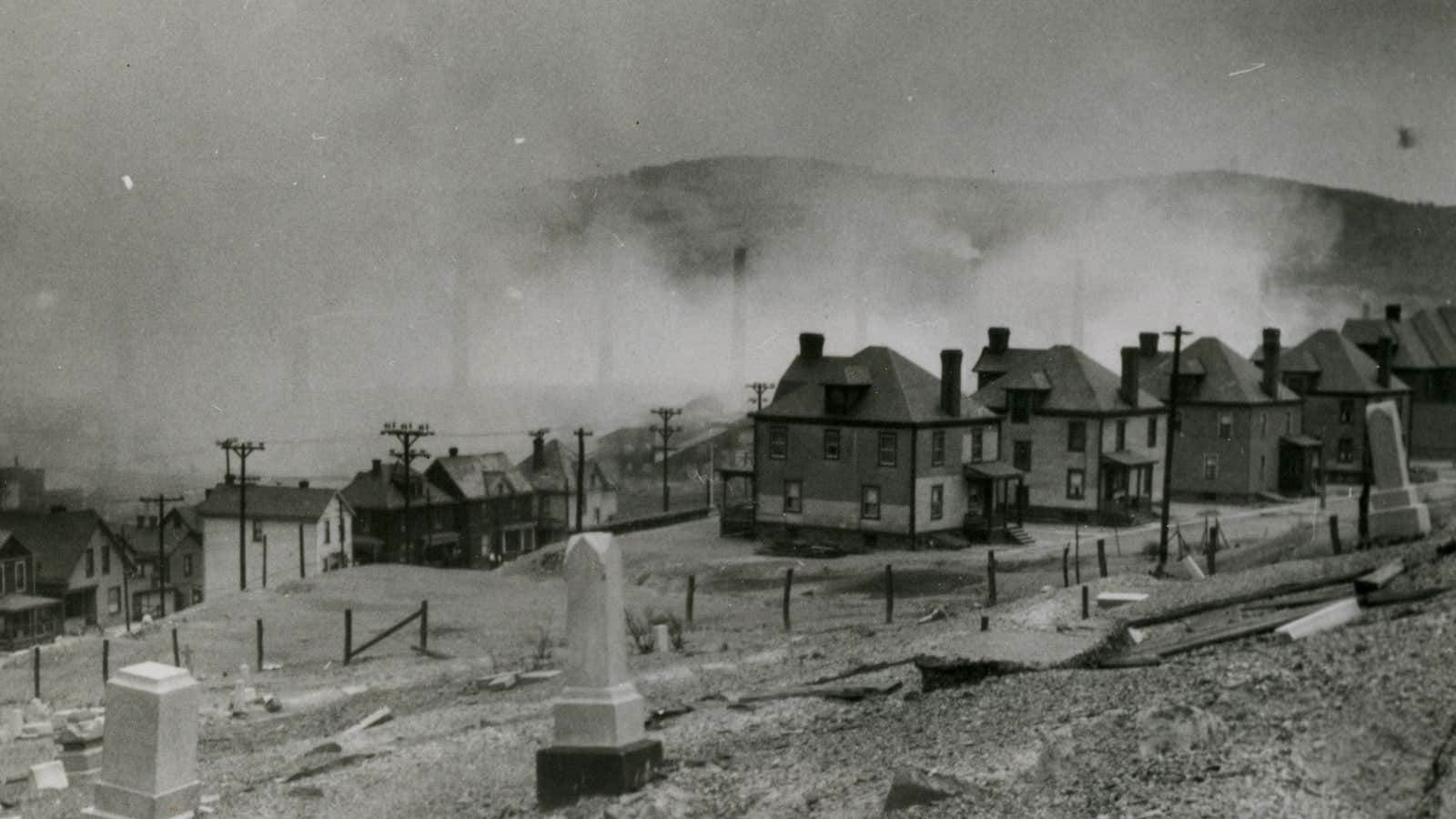This is a black and white photograph with a hint of sepia tone, suggesting its age. The image is taken from a vantage point on a hill, looking down upon a village nestled below. The immediate foreground reveals a graveyard with various headstones, setting a somber tone. In the village, two distinct rows of sizable, two-story row houses are visible, each featuring a square architecture with pyramid-style roofs and chimneys. Some of the houses exhibit slight architectural variations in exterior coloration and material, from brick to light and dark brown hues, adding subtle character to the otherwise uniform structures.

The scene is cloaked in a dense cloud of smoke or dust, likely smoke, given the presence of towering smokestacks in the background, hinting at the village's industrial origins. Electrical poles dot the landscape, marking the era as one where modern amenities were just beginning to take hold. The smokestacks and the pervasive air pollution suggest the village's history is tied to industrial activities, possibly factories or mines, where workers lived in the nearby row houses. 

Further back, the photograph captures either mountains or immense piles of sand or debris, contributing to the eerie and desolate atmosphere that some might mistake for a ghost town during a sandstorm. Makeshift borders or low-lying fences encircle parts of the village, giving an impression of symbolic boundaries rather than functional ones. The overall impression is one of a bygone era, marked by industrial hardship and environmental degradation, encapsulated in this haunting, historic snapshot.